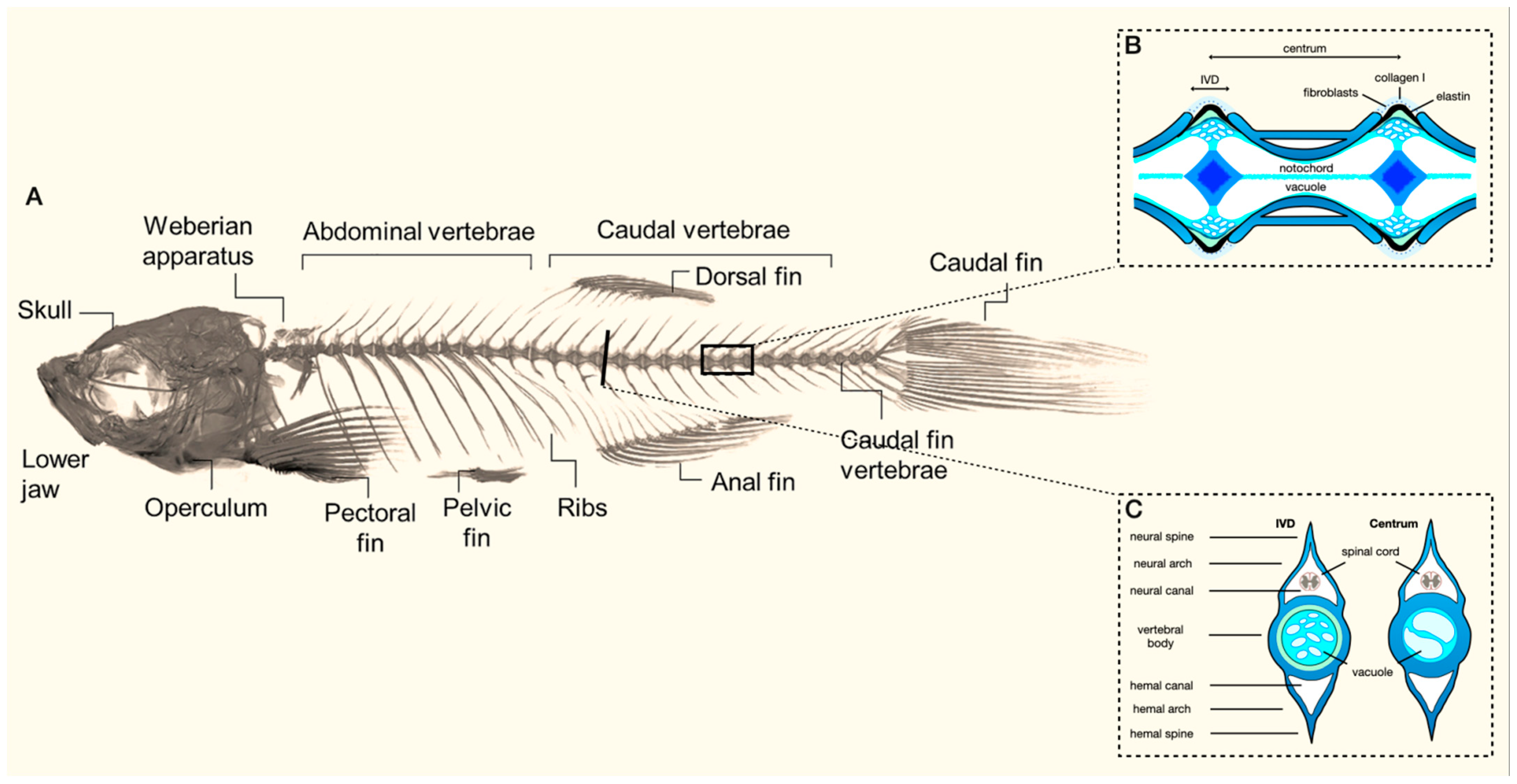This detailed black-and-white graphic showcases the skeleton anatomy of a fish on a very light off-white background. The image meticulously labels various parts of the fish skeleton in black text, including the skull, lower jaw, operculum, pectoral fin, pelvic fin, ribs, anal fin, caudal fin, dorsal fin, caudal vertebrae, abdominal vertebrae, and the web barium apparatus. The skeleton is oriented with the skull facing the left side of the image and the caudal fin extending towards the right. 

Additionally, the graphic features sections labeled A, B, and C on the right side, which include blue diagrams that highlight specific anatomical features such as the spinal cord, neural arch, and neural canal. Section B prominently displays a blue-centered diagram detailing the centrum and fibroblasts. The skeletal elements are outlined with gray and black lines, capturing the intricate structure of the fish in precise detail.

This diagram serves as a comprehensive visual aid to understand the anatomical and biological aspects of a fish skeleton, incorporating complex structures and nerve centers, making it a valuable reference for both general studies and specific inquiries into fish anatomy.